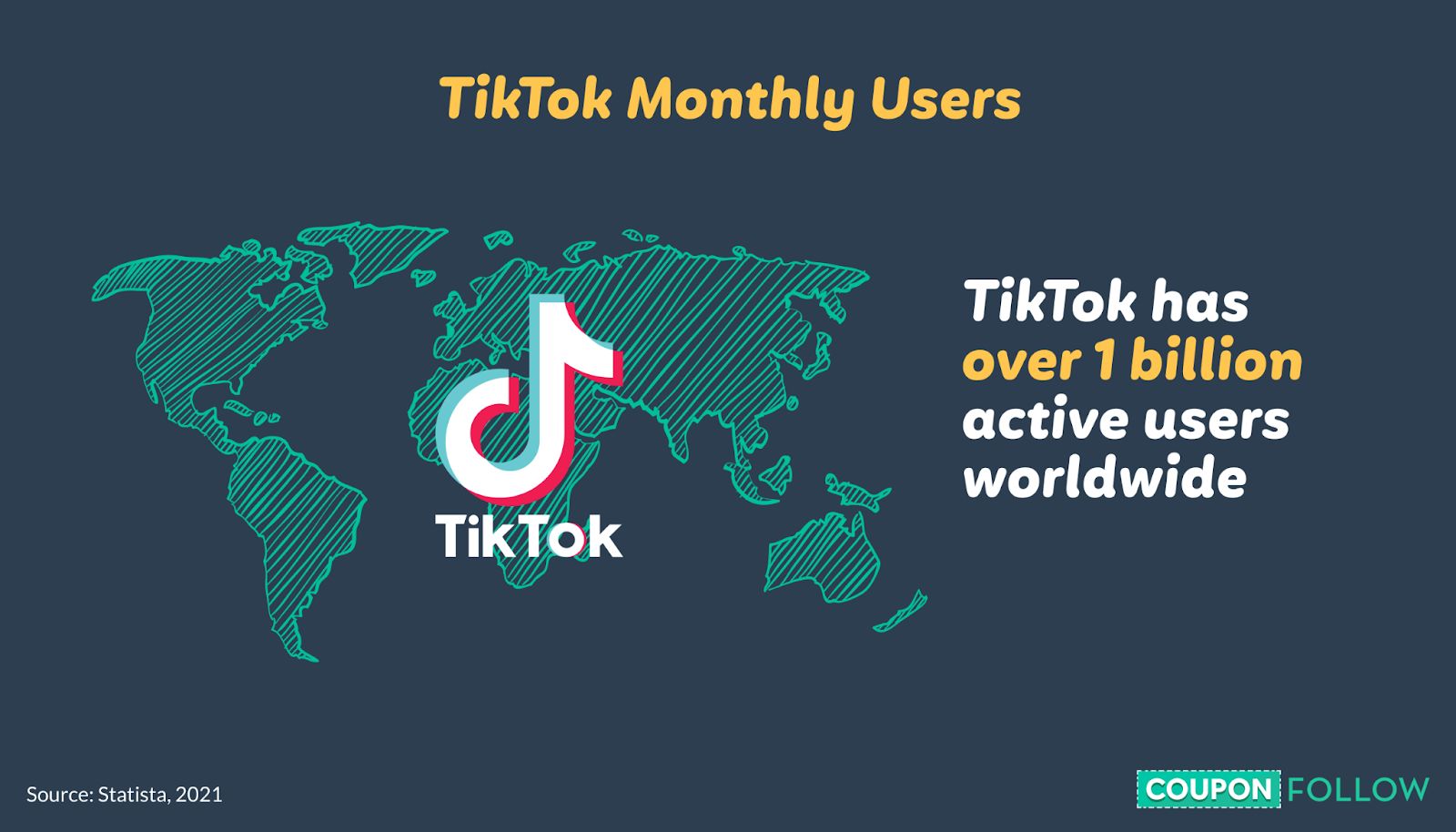The image is a detailed infographic with a dark blue and ghost grey background. In the center, the yellow text "Taz" prominently stands out, signifying its importance. On the lower left corner, the source "Latista 2021" is noted in subtle grey text. On the lower right, a bold blue vertical dash line draws attention to a statistic indicating that TikTok has over 1 billion active users worldwide. Additionally, the image features a map illustrating the global reach of TikTok, accompanied by colorful elements. The TikTok logo is white, surrounded by blue and red accents, contributing to the visual appeal of the infographic. The bottom part of the image includes a call to action with the phrase "Coupon Follow," enhancing its interactive nature.